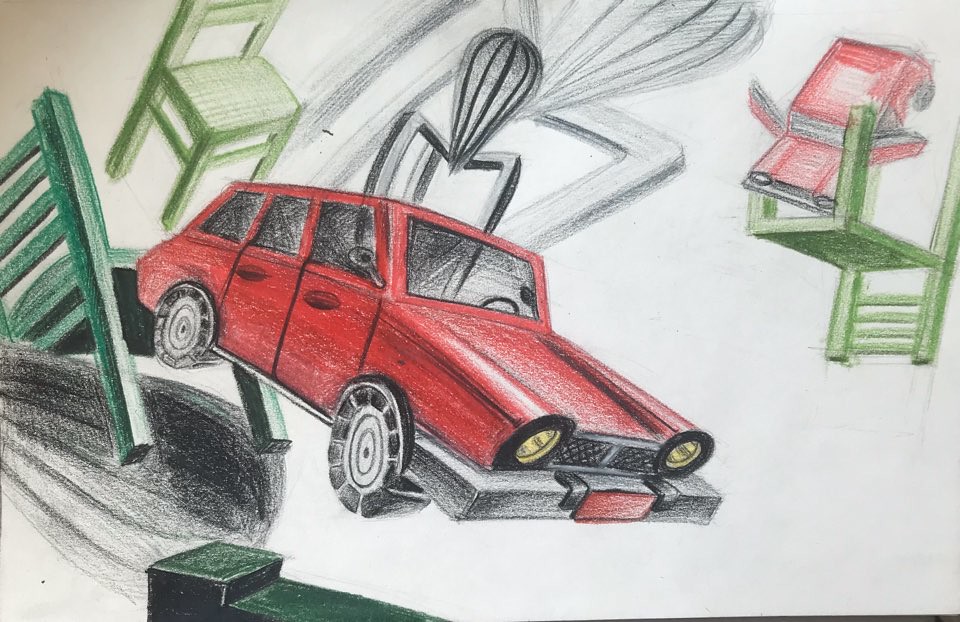In this vibrant colored pencil drawing, the central focus is a vintage red car, reminiscent of models from the 1970s or 1980s, being lifted by the mechanical claw of a whimsical claw machine. The background is set against a stark white paper, highlighting the intriguing scene. Behind the claw-clutched car, a larger-than-life claw machine looms, amplifying the fantastical nature of the artwork. To the left, a peculiar green chair perches atop a floating blimp, adding an eccentric flair. In the distant background, another green chair can be glimpsed. On the right side of the drawing, a smaller or more distant version of the same red car appears to be either falling into or riding towards a large, inverted green chair, further adding to the surreal and dreamlike composition of the piece.